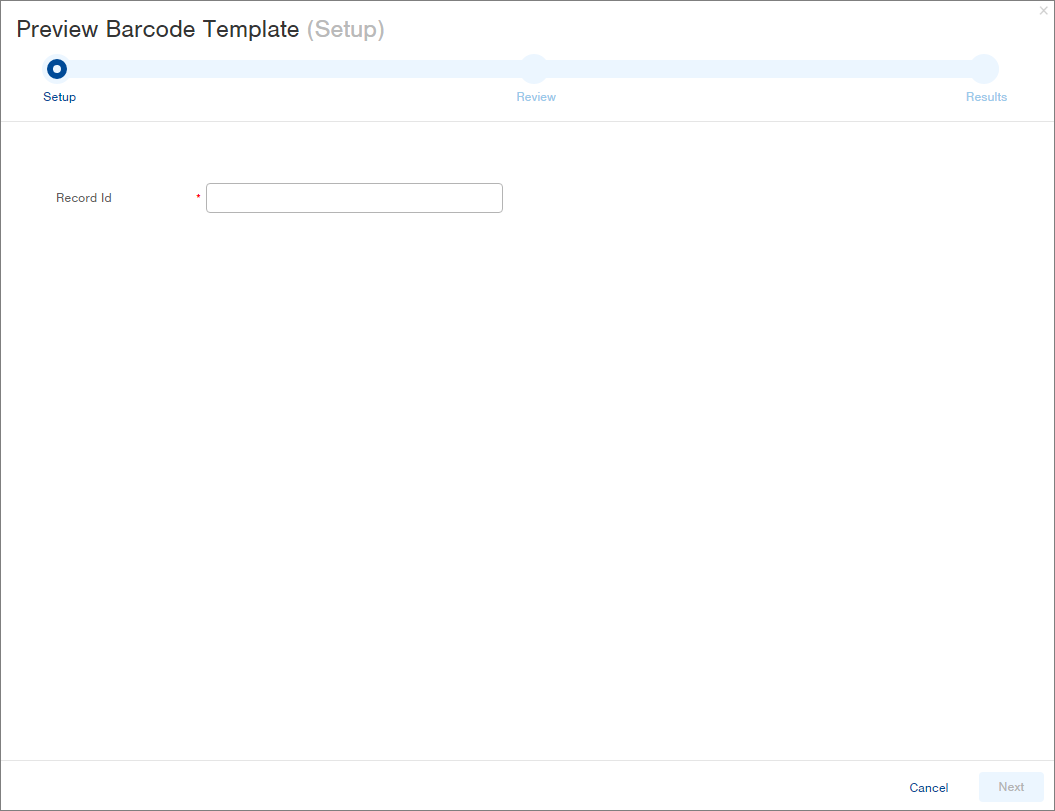This image depicts a web interface page with a minimalist design, characterized by a significant amount of white space and minimal textual content. The main layout is a rectangular section bordered in either dark grey or black. The background of this section is predominantly white.

In the upper left-hand corner of the rectangle, there are the words "Preview," "Barcode," and "Template," each starting with a capital letter and in black text. Following these words, in light grey, is "Setup" with a capital 'S'.

Below this, there is a blue progress bar running horizontally. A dark blue circle with a hole in the middle indicates progress within this bar, showcasing the underlying light blue. The progress bar appears to have three segments, each labeled with a step name: "Setup" (currently highlighted in dark blue), "Review" (in lighter blue), and "Results" (also in lighter blue).

Beneath this progress bar, text in black reads "Record ID," with "Record" and "ID" both capitalized. Adjacent to this text is a rectangular input box, white inside with a black border, marked by a red asterisk indicating a required field.

At the bottom of the rectangle, a thin grey line spans horizontally, followed by two buttons: "Cancel" in blue text, and a blue button labeled "Next" written in grey.